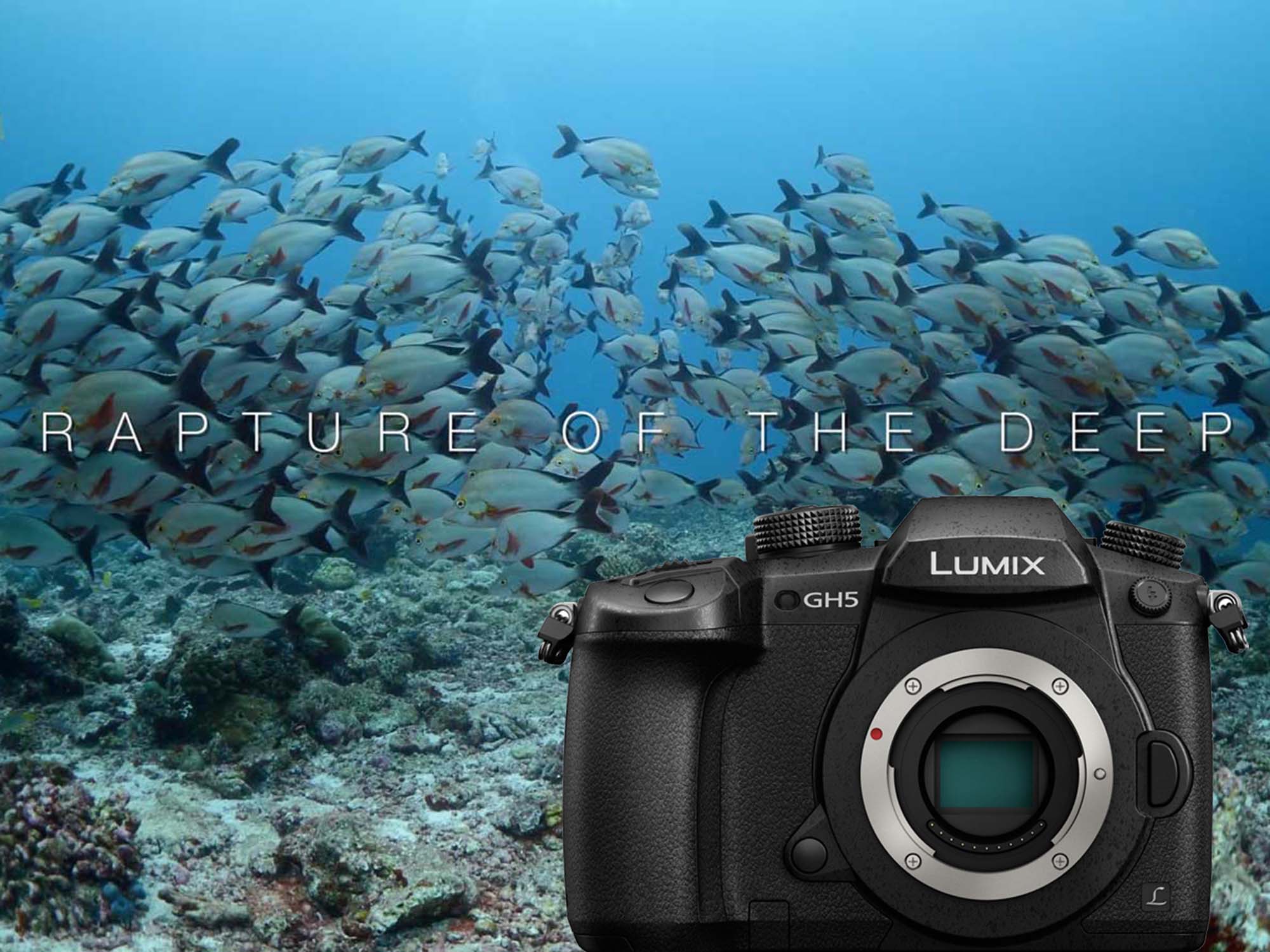The advertisement features a Lumix GH5 camera prominently in the foreground, showcasing its sleek black body accented by a silver ring around its greenish lens. Notable design elements include knurled knobs on the top and a textured grip. The backdrop is an underwater scene teeming with life, highlighted by a school of oblong fish with white bodies and dark tails, moving in opposite directions. The vibrant blue ocean envelops scattered lichens and shells, adding depth to the serene environment. Stretching across the center of the image, the phrase "Rapture of the Deep" is emblazoned in bold white letters, drawing attention to the immersive aquatic setting. The camera, in the left-hand corner, faces the viewer, standing out amidst the lively marine backdrop.